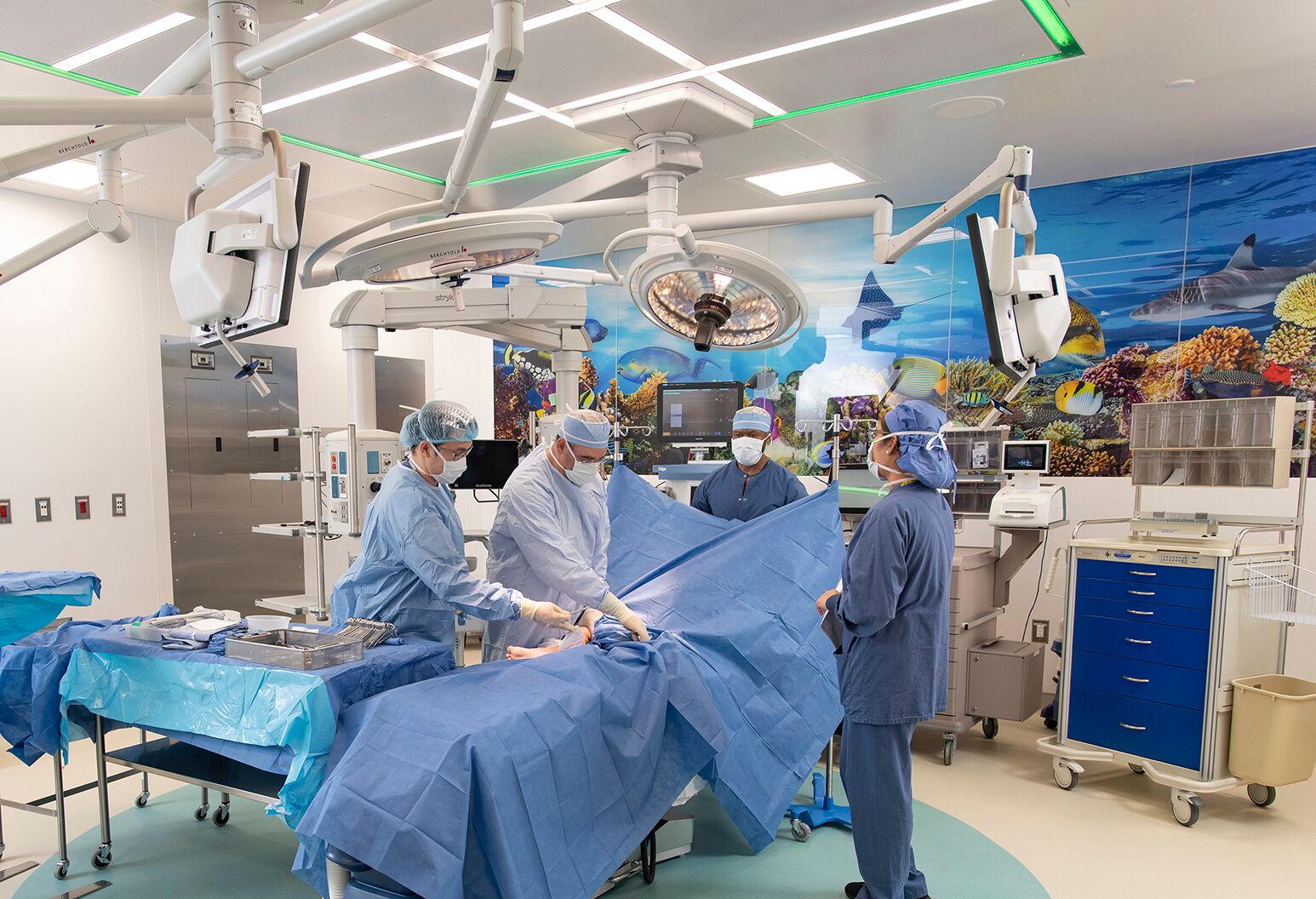This detailed photograph captures the interior of an operating room in what appears to be a hospital, possibly designed with children in mind, given the prominent, colorful mural depicting a realistic coral reef with blue waves, tropical fish, and coral, which adorns one wall behind the patient. The room is brightly lit with several overhead surgical lights, sterile white fixtures, and a distinctive white floor marked by a large aqua blue circle in the center. A patient, covered with blue surgical drapes, lies on the operating table, surrounded by four medical professionals dressed in scrubs, hats, and face masks. Two surgeons are positioned on the left side of the patient, apparently engaged in the procedure, while another stands behind the patient. A fourth person is situated on the right side of the photograph, appearing to monitor or assist with the operation. The scene also features a variety of medical equipment, including an instrument table with blue sheets covering surgical tools and a rolling cart. The dominant color palette of the room, aside from the vibrant mural, is primarily blue and white, contributing to the sterile but serene atmosphere typical of an operating theater.